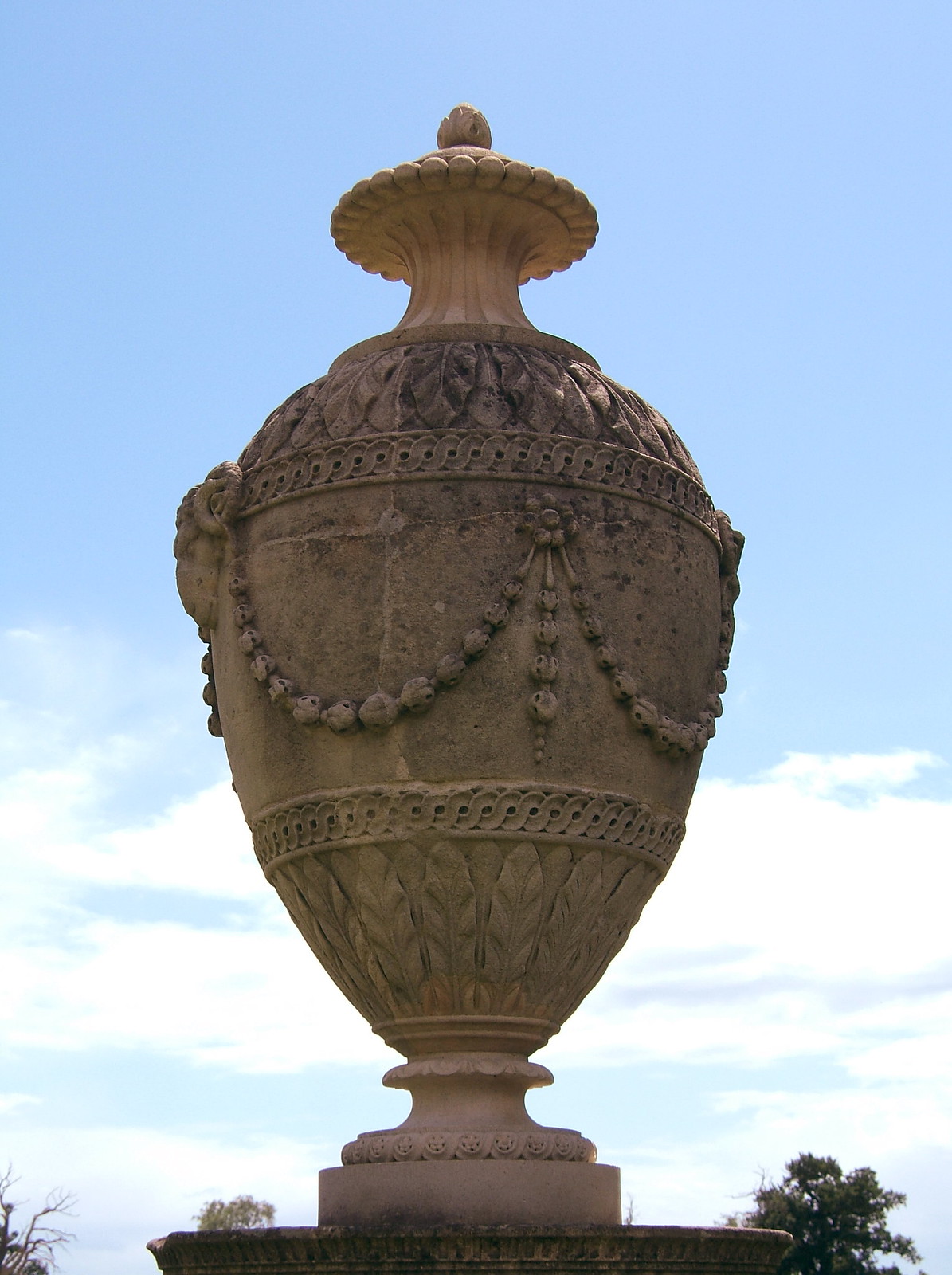The photograph captures an intricate, egg-shaped stone sculpture set against a vivid daytime sky. The sculpture, which resembles an inverted urn or a vase, is mounted on a round, ornately-carved base. Its surface is adorned with carved garlands, feathers, and beads, leading up to a mushroom-shaped top adorned with multiple small spheres around the edge and culminating in a round, plant-like finial. The backdrop reveals a light blue sky gradually transitioning to a canvas interspersed with white and light gray clouds. Peeking from the bottom, the tops of lush green trees frame the scene, with varying foliage density contributing to the tranquil ambiance.